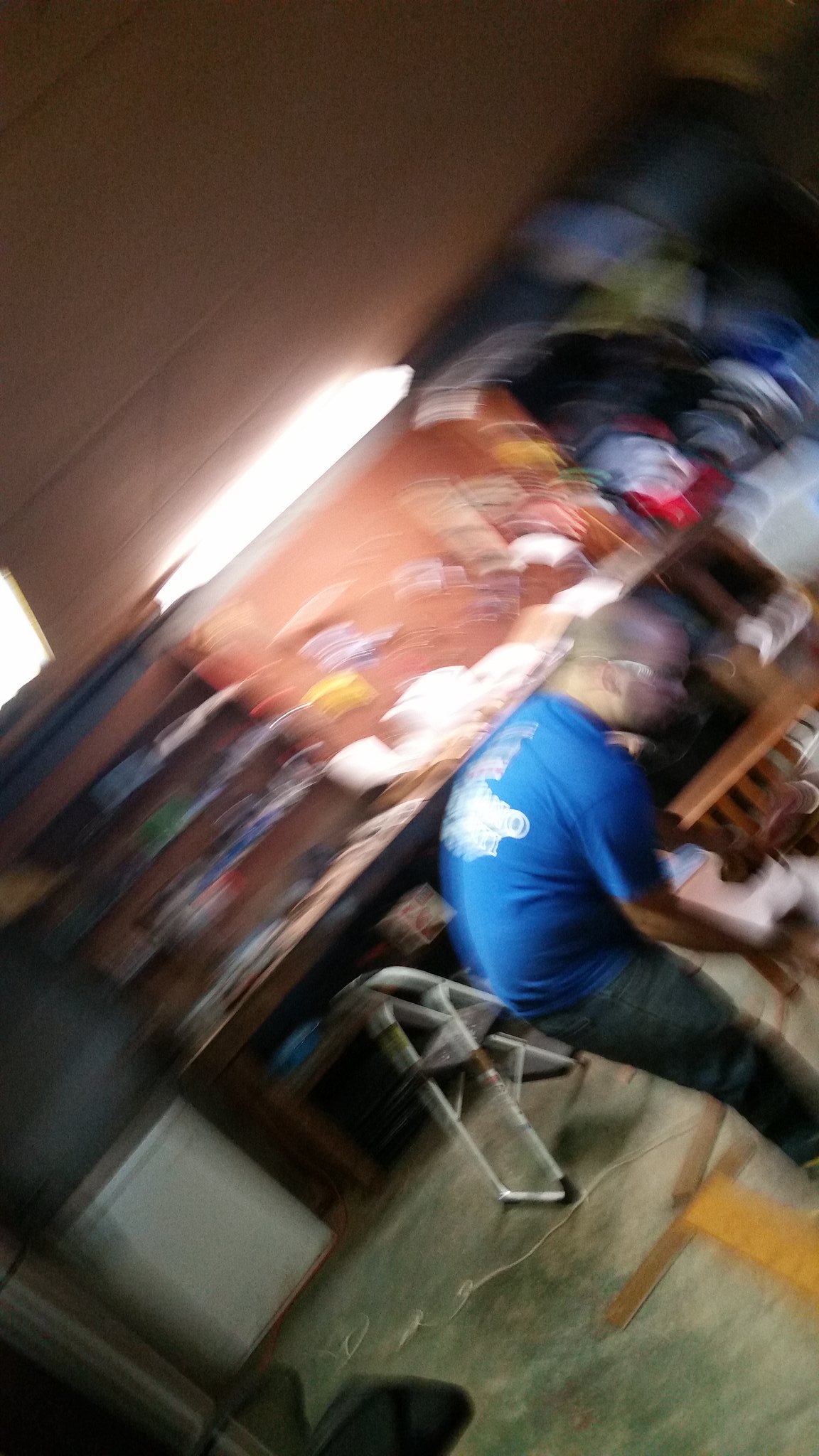This photograph captures a somewhat chaotic scene in what appears to be a workshop or garage, characterized by its noticeable blur and a pronounced tilt to the right, suggesting the camera was moved suddenly, resulting in a dynamic, off-kilter composition. Central to the image is a gentleman in a blue short-sleeved t-shirt with a white logo on the back, and blue jeans, who is bent over at the waist, possibly working on a desk or table. The floor beneath him is concrete, scattered with pieces of wood, reinforcing the workshop environment. In the background, there are shelves running along the length of the wall, cluttered with indistinguishable items due to the motion blur. A workbench is also visible at the back, potentially illuminated by a large light, with a pegboard adorned with hanging tools. Additionally, a white and black stepstool is placed on the concrete floor, further emphasizing the utilitarian nature of the space. The overall blur, whether accidental or intentional, adds a sense of urgency and movement to the scene.